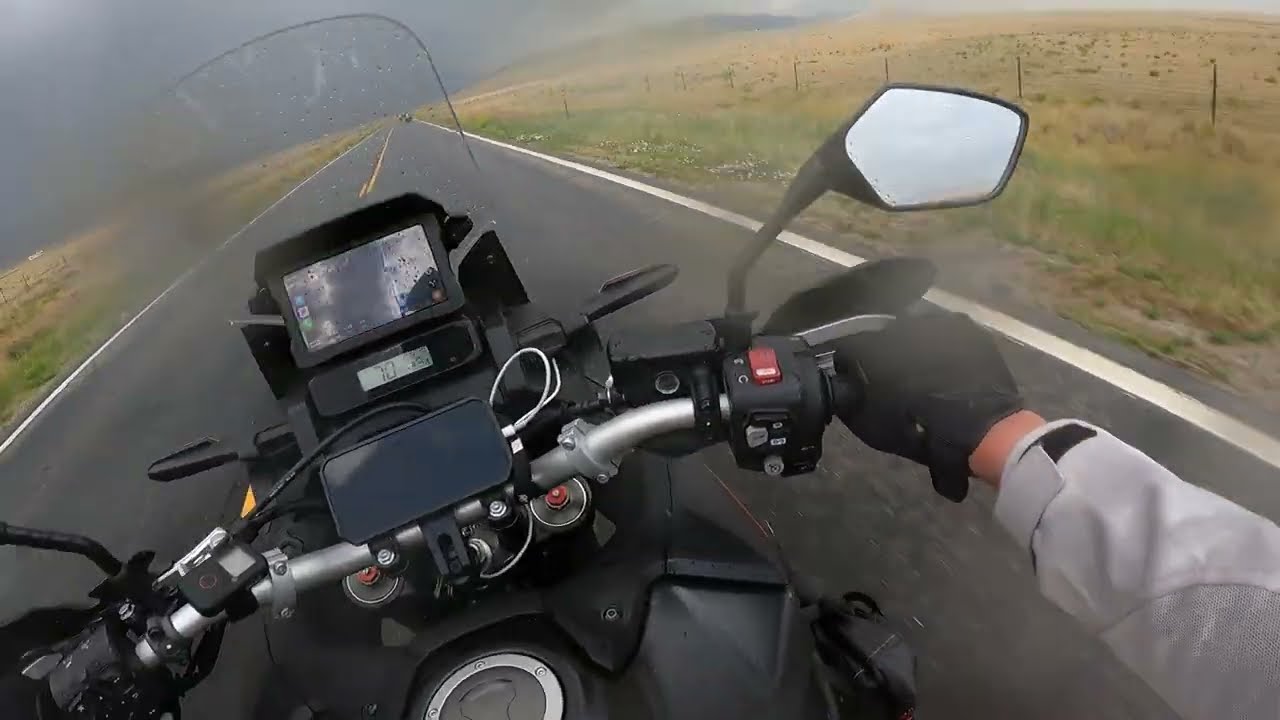The image captures a first-person perspective from a motorcycle, likely taken from a helmet-mounted camera. The view showcases a motorcyclist's right hand, clad in a black glove, gripping the handlebars. The rider is wearing a gray coat with a Velcro strap on the sleeve. The motorcycle features a cell phone mounted centrally on the handlebars, positioned slightly behind a smaller screen displaying a temperature reading of 70 degrees. Additional gadgets are also visible on the handlebars. There are rear-view mirrors and a small clear windshield above the secondary screen. Raindrops are noticeable on the screens, mirrors, and windshield, indicating that it is raining. The motorcycle is traveling on the right side of a two-lane road in a rural area, with open fields and grassy areas flanking the highway. In the background, faint hills and a distant vehicle on the same lane are visible under a cloudy sky, with some dust apparent in the scene.